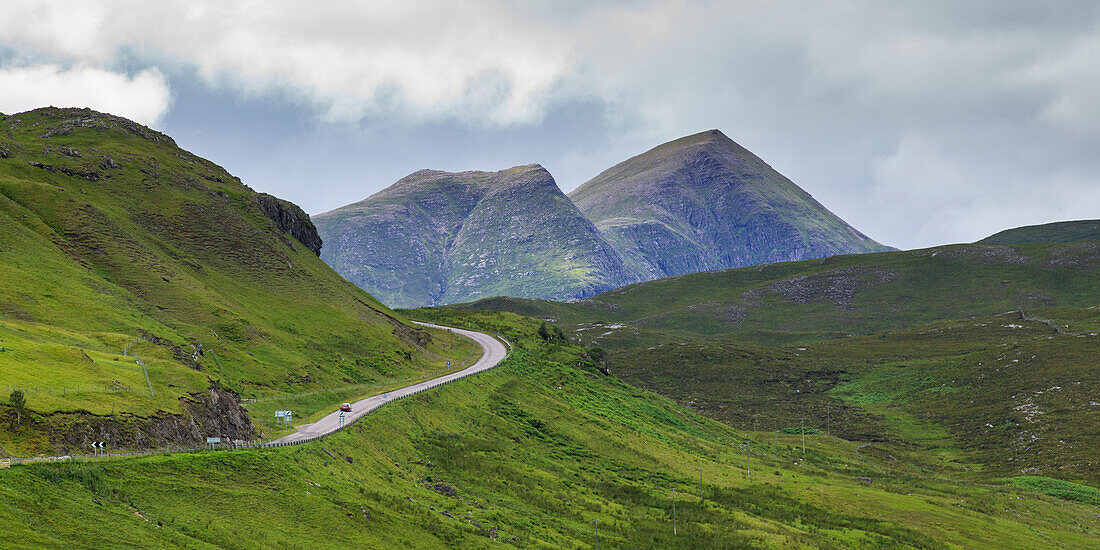The image portrays a stunning landscape with vibrant details. Dominating the scene is a central mountain, partially covered in grass with visible brown patches. This mountain is flanked by a lush green valley to the right, dotted with bushes and stretching clear fields, while a similar hill rises to the left, also marked by patches of green grass and brown dirt. A well-maintained gray road snakes through the landscape, hugging the left hill where a red car can be seen driving. A silver guardrail lines the road, accompanied by a fence. Further accentuating the scene are distant mountain ranges in the middle background, exhibiting a blue hue over their brown and tan surface, adding depth to the photograph. Above, a serene blue sky dotted with fluffy white clouds blankets the picturesque view. The overall scene is a harmonious blend of natural beauty and man-made elements, capturing the essence of a tranquil countryside journey.